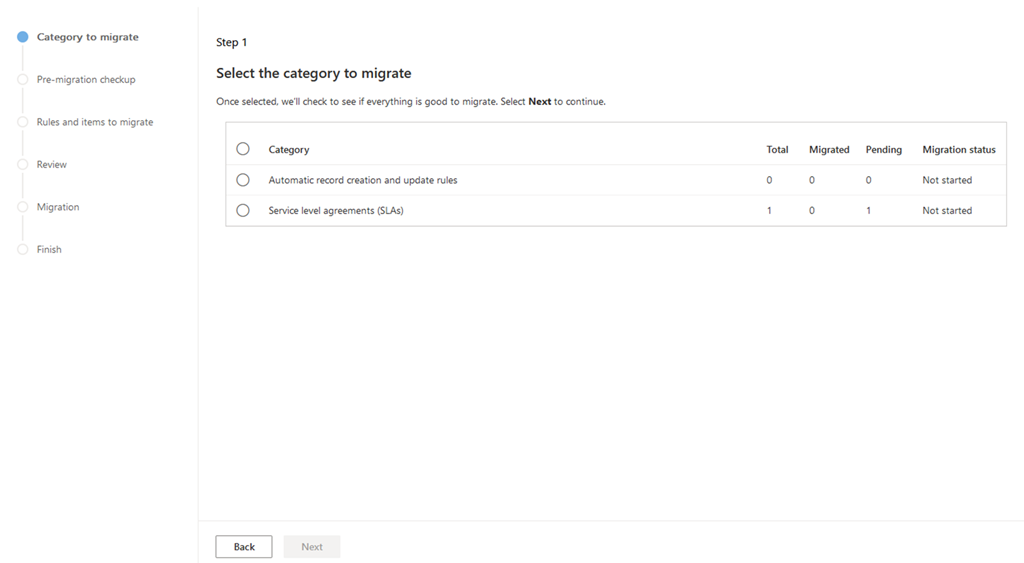### Image Caption: Detailed Migration Process Overview

The image illustrates a step-by-step process for data migration, represented by a series of connected stages. 

1. **Category to Migrate**: Indicated by a blue dot, this is the initial step where you select the data category to be migrated.
2. **Pre-migration Checkup**: Marked by a line followed by a white dot, this step ensures that the selected category is ready for migration. Any issues are flagged for correction.
3. **Rules and Items to Migrate**: Another line and white dot denote this phase, where specific rules and items to be migrated are identified.
4. **Review**: Following another line and dot sequence, this stage involves a thorough review of the selected items and rules to ensure accuracy.
5. **Migration**: Marked by an additional line and dot, this step initiates the actual migration of data.
6. **Finish**: The final stage, indicated by a line and dot, signifies the completion of the migration process.

Below the main steps, there's additional information:
- **Automatic Record Creation and Update Rules**: Displaying a circle next to the category for setting rules regarding data records.
- **Service Level Agreements**: This section has a circle next to it indicating considerations for service agreements during migration.
- **Summary Panel**: Shows total items (0 of 1), migrated items (0 of 0), and pending items (0 of 1), with a status indicating "Migration Not Started."

At the bottom of the interface:
- **Back Button**: Allows you to return to the previous step.
- **Next Button**: Initially grayed out until the necessary steps are completed to proceed further.

Note: The voiceover ends with a personal message to the speaker's mother, indicating their love and reassurances, but this part is unrelated to the data migration process.